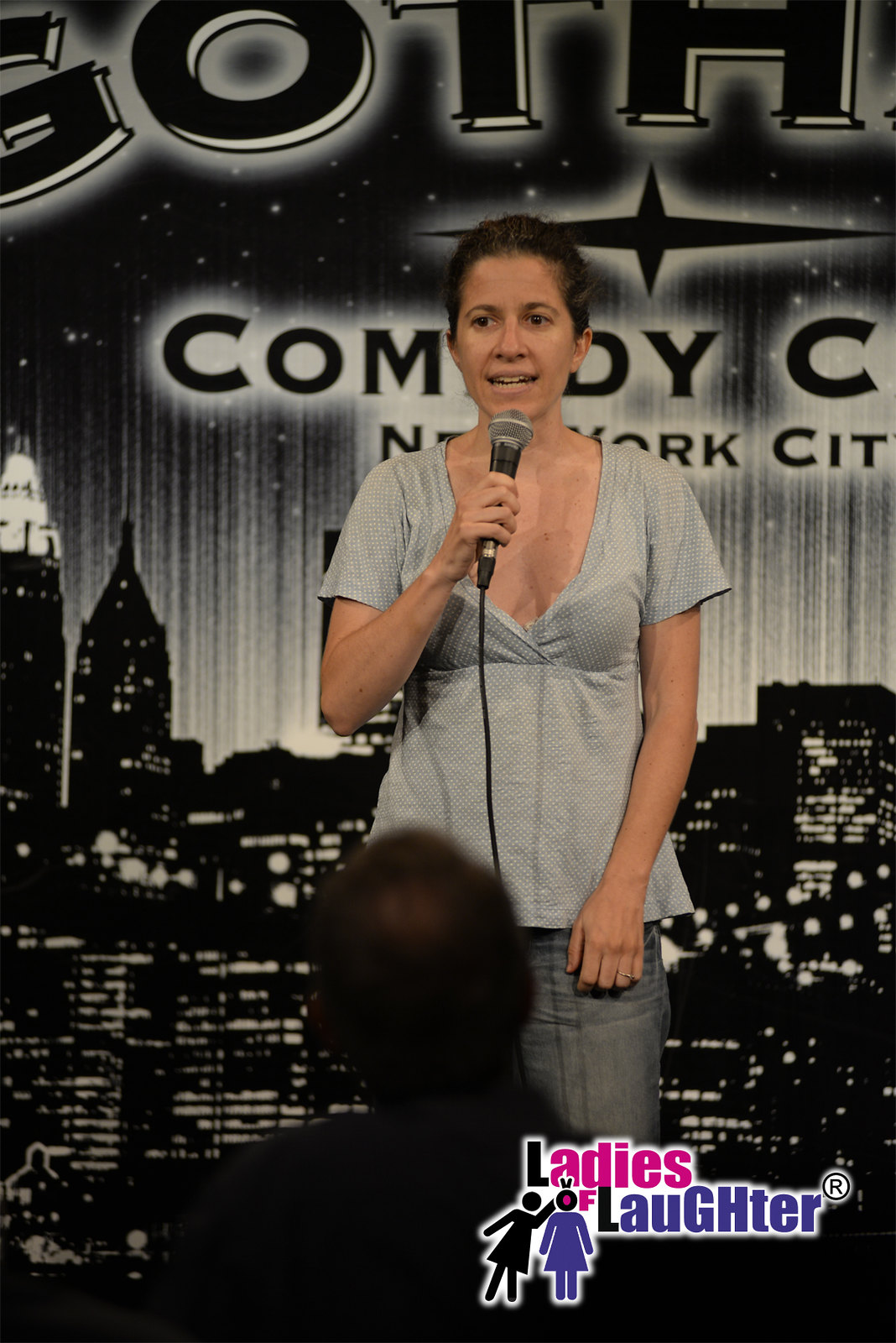A woman, dressed in a gray short-sleeved tunic with a deep V-neck and jeans, is performing a stand-up comedy routine at the Gotham Comedy Club in New York City. She has dark brown hair, swept back, possibly in a bun or ponytail. The background features the club's signature black-and-white cityscape, depicting New York City's illuminated skyscrapers at night. Partially visible text above her reads "GOTH" and "Comedy Club New York City." At the bottom of the photo, the colorful words "Ladies Laughter" stand out, with "Ladies" in pink, "Laughter" in purple, and both "L" letters in black, accompanied by two stick figure women.